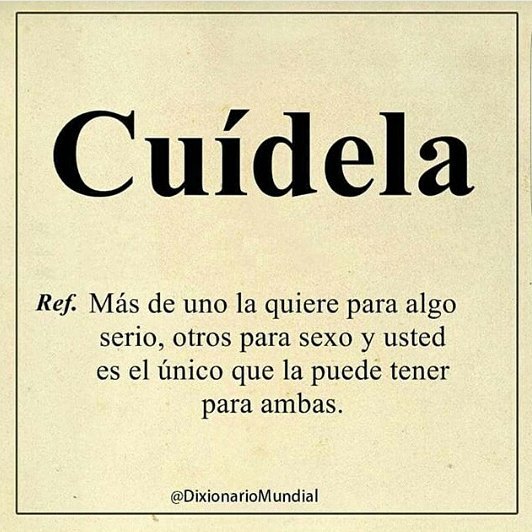This square graphic, designed possibly for social media or web posting, features a cream-colored, beigey pink background with a thin black borderline framing the outer edges. Dominating the center in bold, large black letters is the word "Cuidela" (C-U-I-D-E-L-A). Below it, in smaller black text, is the abbreviation "R-E-F." At the image's base is a smaller text handle reading "Ad Diccionario Mundial." The neat, contrasting colors and clear typography make it a visually striking and easily shareable piece.